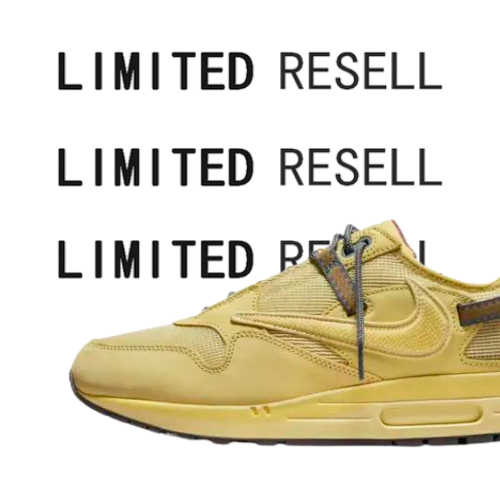The image features a mustard-colored Nike sneaker set against a solid white background. Positioned along the bottom of the image with its toe facing left, the shoe’s back end is slightly cut off by the left edge. This Nike sneaker has a backwards-facing Nike swoosh in the same mustard hue and darker brown patches accentuating the areas around the laces and sides. The laces are dark gray, possibly black, and one is hanging down untied. The tan-colored sole has a thin black layer at the very bottom. Three left-aligned lines of text in black capital letters appear above the shoe: "LIMITED RESELL," "LIMITED RESELL," and "LIMITED RESELL," with the bottom line partially obscured by the sneaker. The word "LIMITED" is bolded in each line, while "RESELL" is in regular font.